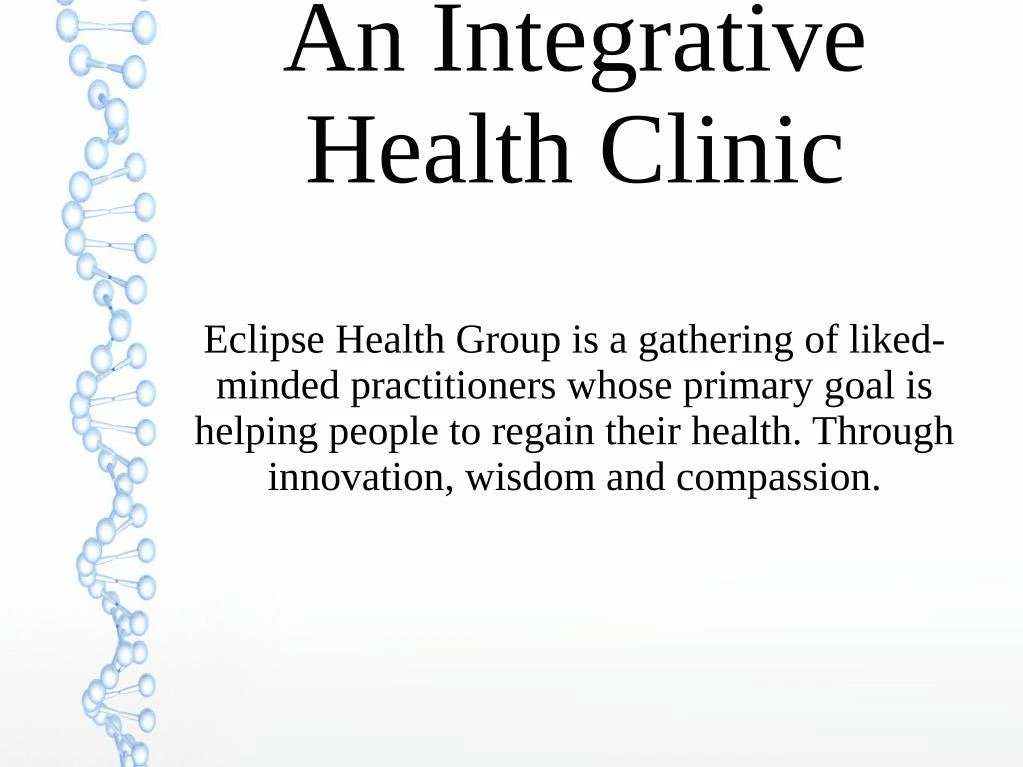The image is an information graphic, likely a PowerPoint slide or presentation type of slide, designed with a clean, white background. Dominating the left side is a light powder blue sketch of a DNA double helix, rendered in a wireframe style. Each side of the helix is composed of small blue circles connected by rod-like shapes. At the top of the image, in a large bold serif font, is the title "An Integrative Health Clinic," with each word capitalized. Below the title, in smaller text, there is a paragraph that reads: "Eclipse Health Group is a gathering of like-minded practitioners whose primary goal is helping people to regain their health through innovation, wisdom, and compassion." It should be noted that there is a typographical error in the text; it incorrectly reads "liked-minded" instead of "like-minded." Overall, the graphic conveys a welcoming message that is likely intended for a medical facility, emphasizing a mission of health recovery through innovative and compassionate practices.